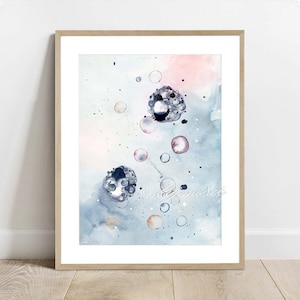On a light wood floor, against a white wall with a white baseboard, stands a thin, rectangular, pale brown wooden frame. The frame contains a piece of abstract art that features a white matte board. The artwork itself appears like a dreamy watercolor composition with a soft, fuzzy background blending shades of light blue, white, and light pink. Delicate, large, gem-like shapes in black and white create an organic, bubbly texture across the image, interspersed with various-sized water droplets and fine black specks. The subtle hues and layered circular forms lend it a 3D effect, making the entire piece enigmatic and visually intriguing.